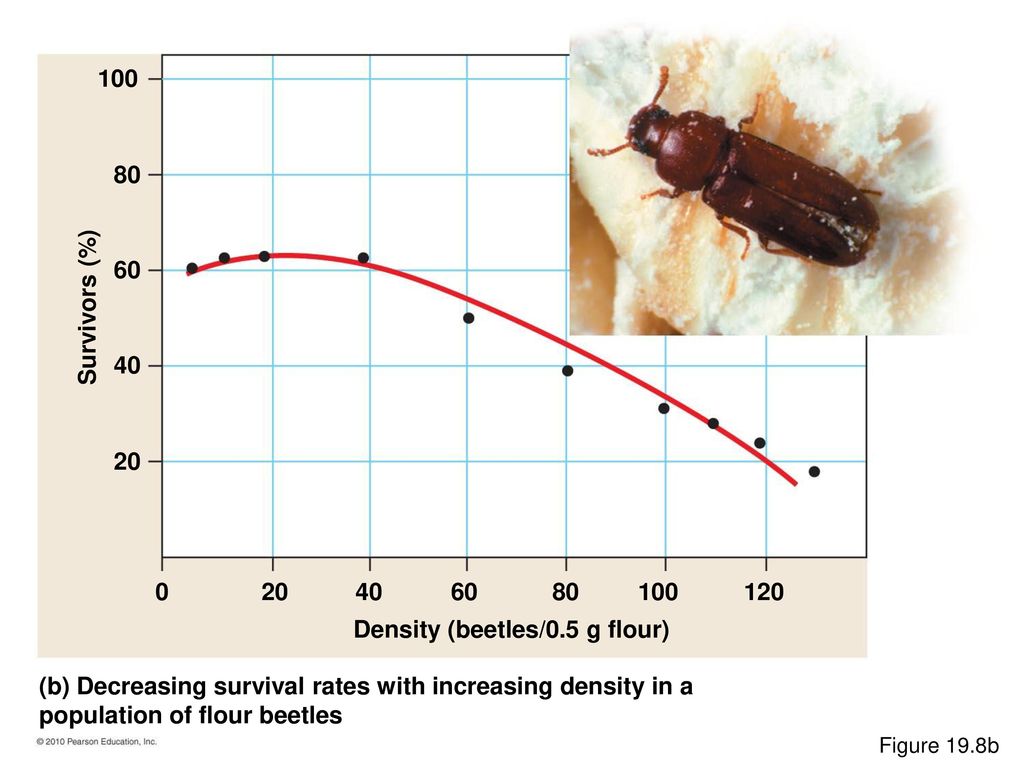The image features a detailed graph displaying the relationship between the survivability of flower beetles and their population density. The graph is set against a brownish-grayish backdrop and features white grid lines. On the y-axis, labeled "Survivors (%)", the scale ranges from 0 to 100 in increments of 20. On the x-axis, labeled "Density (beetles per 0.5 grams of flour)", the scale ranges from 0 to 120. The trend line suggests that as the density of beetles increases, the survival rate decreases. Below the graph, a caption reads: "Decreasing survival rates with increasing density in a population of flower beetles." 

In the upper right corner of the image, an inset photo displays a close-up of a flower beetle on a piece of flour, emphasizing the context of the graph. Despite its placement, the beetle photo does not obscure the trend line on the graph. The overall image effectively illustrates the inverse relationship between population density and survivability in flower beetles.